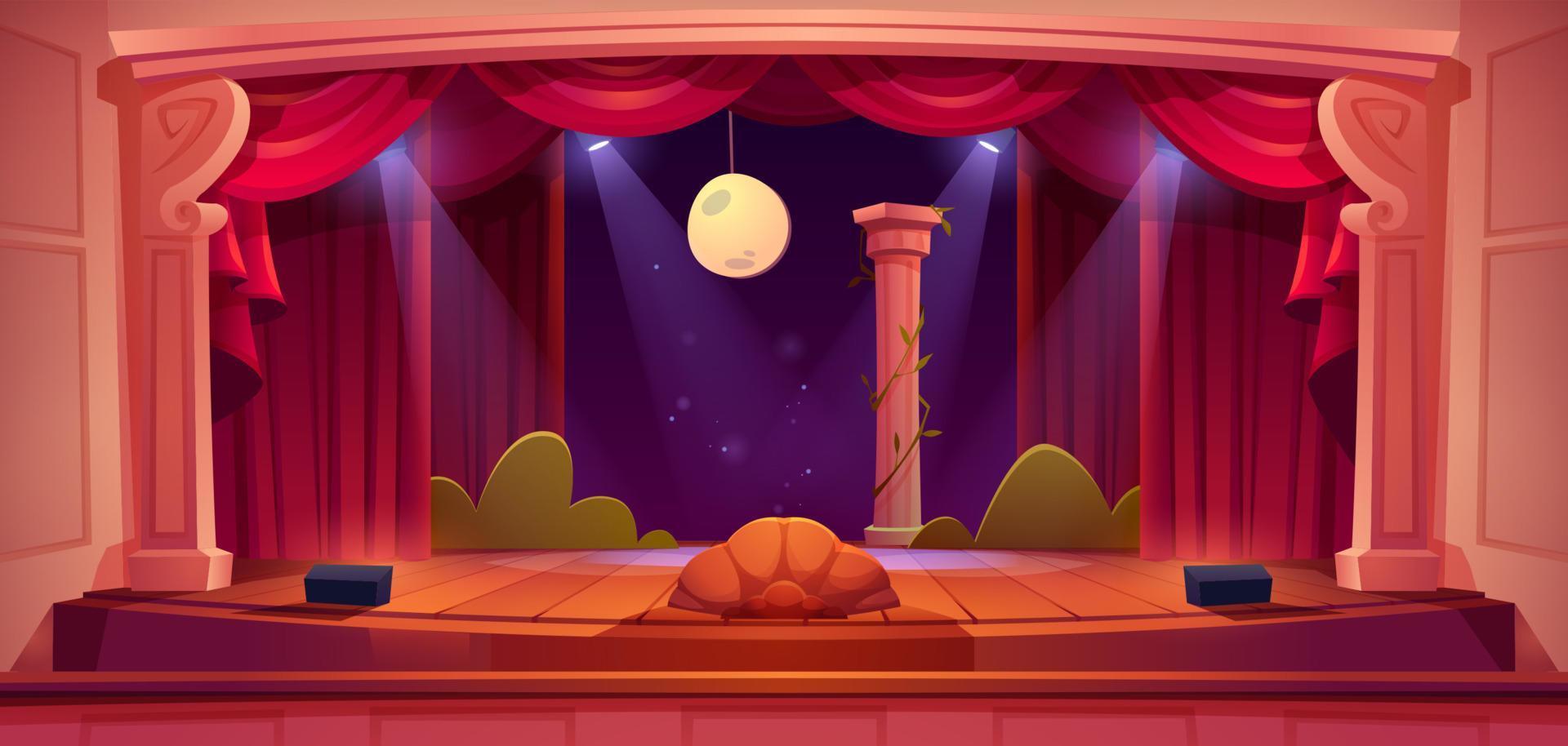The image depicts an elaborate, cartoonish mock-up of a theatrical stage set, characterized by its vibrant colors and stylized, rounded objects. The stage is flanked by faux columns on either side, evoking a classical Greek or Roman aesthetic, and is topped by a pinkish-red draped curtain, flounced grandly along the upper edge. Behind this main curtain, two additional sets of red pleated curtains add depth to the scene. In the foreground, the orange stage floor features a prominent scalloped or shell-shaped central prop, flanked by four visible speakers or stage footlights—two in the forefront and two more outlined by their beams. Soft mounds of green, indicative of bushes or trees, are positioned towards the back, contributing to the whimsical atmosphere. The backdrop comprises a blue panel adorned with stars and a dangling moon suspended from a string, enhancing the fantastical environment. An ornamental purple column, entwined with green vines, stands prominently at the rear, completing this enchanting stage set. Notably, the context of the play or performance remains a mystery, as there are no visible characters or text to provide further clues.